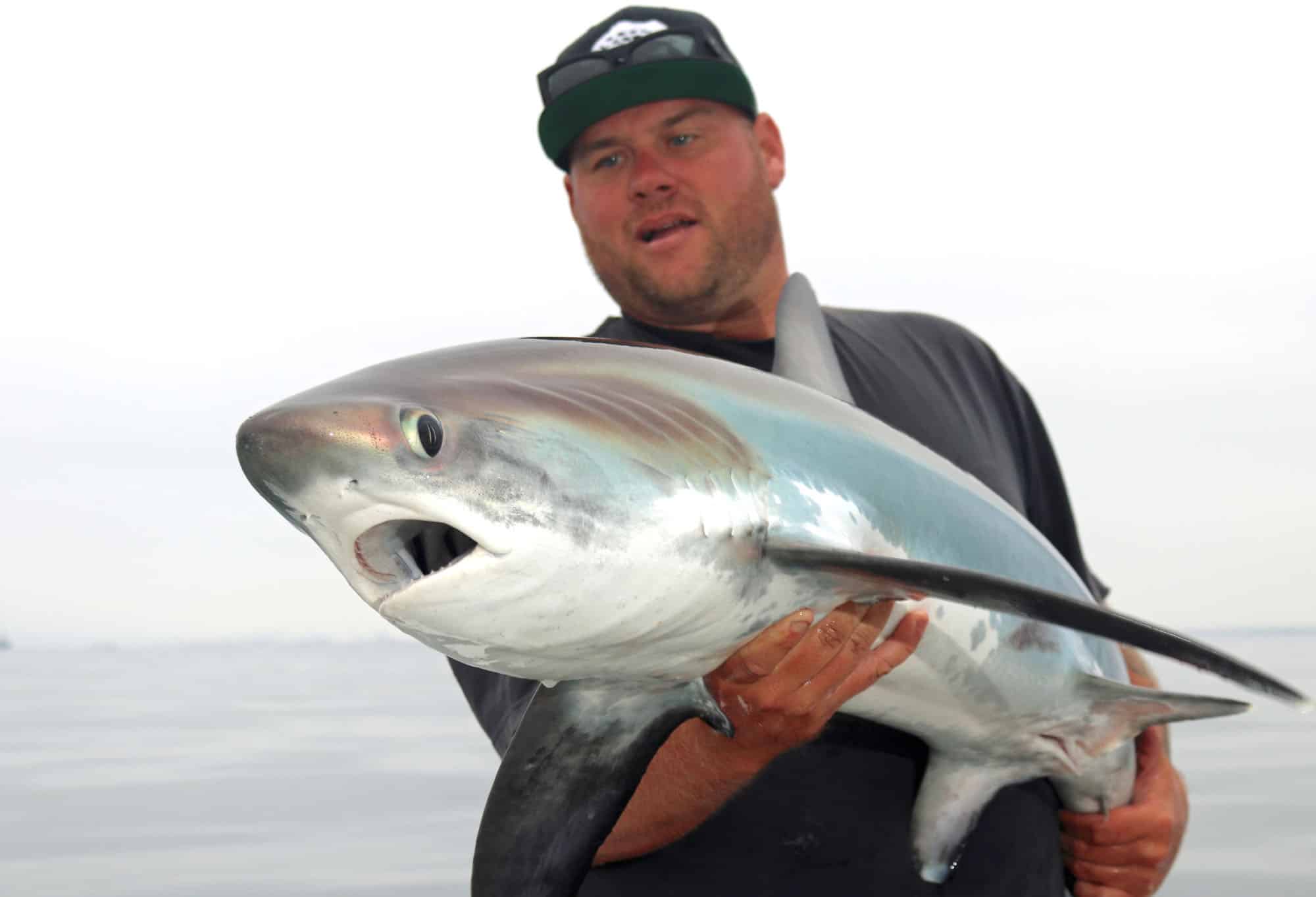In the photograph, a slightly stout man with stubble is seen from the waist up, standing near the center of the image and holding a small shark. He is dressed in a short-sleeved, dark T-shirt and a black baseball cap with a green rim, upon which a black-framed pair of sunglasses rests. His right hand is positioned under the belly of the shark, just behind its side fin, while his left hand grasps the tail. The shark, roughly the size of the man's torso, is oriented to the left and slightly forward, showcasing its gray, silver-hued top and white underbelly. Its open mouth reveals small pointed teeth, and it has prominent black eyes and nostrils on its conical snout. Both sides of the shark display darker gray gills. The backdrop reveals a vast blue body of water beneath a light gray sky filled with darker gray clouds.